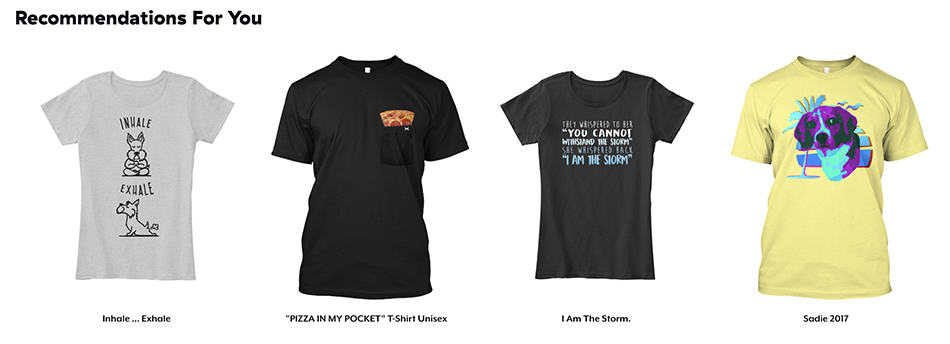This is a sale page featuring personalized recommendations for you. 

1. The first recommendation is a women's gray scoop-neck t-shirt. The sleeves are cut in a way that indicates it is designed for women. The shirt features an illustration of a dog at the top sitting cross-legged with the text "inhale." At the bottom, the same dog is stretching out with the text "exhale."
   
2. The second recommendation is a unisex black t-shirt with a pocket. Peeking out from the pocket is the crust end of a pizza slice, and the shirt is labeled "Pizza in my Pocket T-shirt."
   
3. The third recommendation is another black t-shirt with a bold statement. It reads, "When someone tells you you cannot withstand the storm, you whisper back, 'I am the storm.'"
   
4. The final recommendation is a yellow t-shirt featuring a stylized image of a beagle. Interestingly, the dog's colors are unconventional, rendered in purple, black, and white instead of the traditional beagle colors.